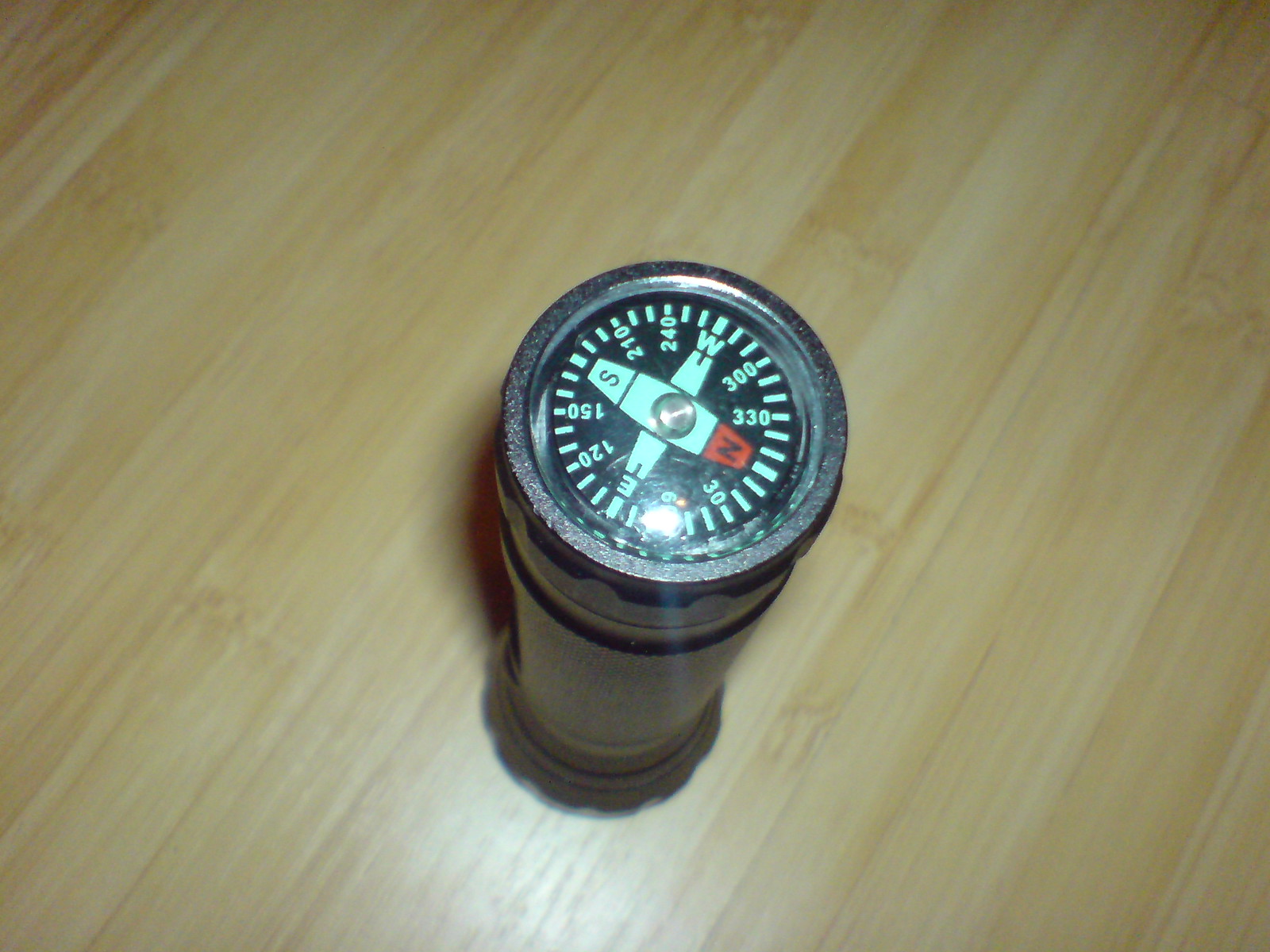In this square-shaped photograph, the focal point is a black, metallic, tube-shaped object centrally positioned on a light brown table. The table appears slightly darker in the top left and top right corners. The image is captured from an overhead perspective, showing the object standing vertically.

At its base, closest to the table, the object features a ridged, circular component that suggests it might be adjustable or equipped with dials. Extending upwards from the base is a smooth, black, cylindrical shaft leading to the top section, which also has ridges around its edge. The centerpiece of this top section is a compass. The compass face is predominantly sea green, with cardinal directions marked clearly: north indicated in red, and west, south, and east also labeled. The compass is detailed with additional coordinates, providing a functional and aesthetic element to the metallic object.